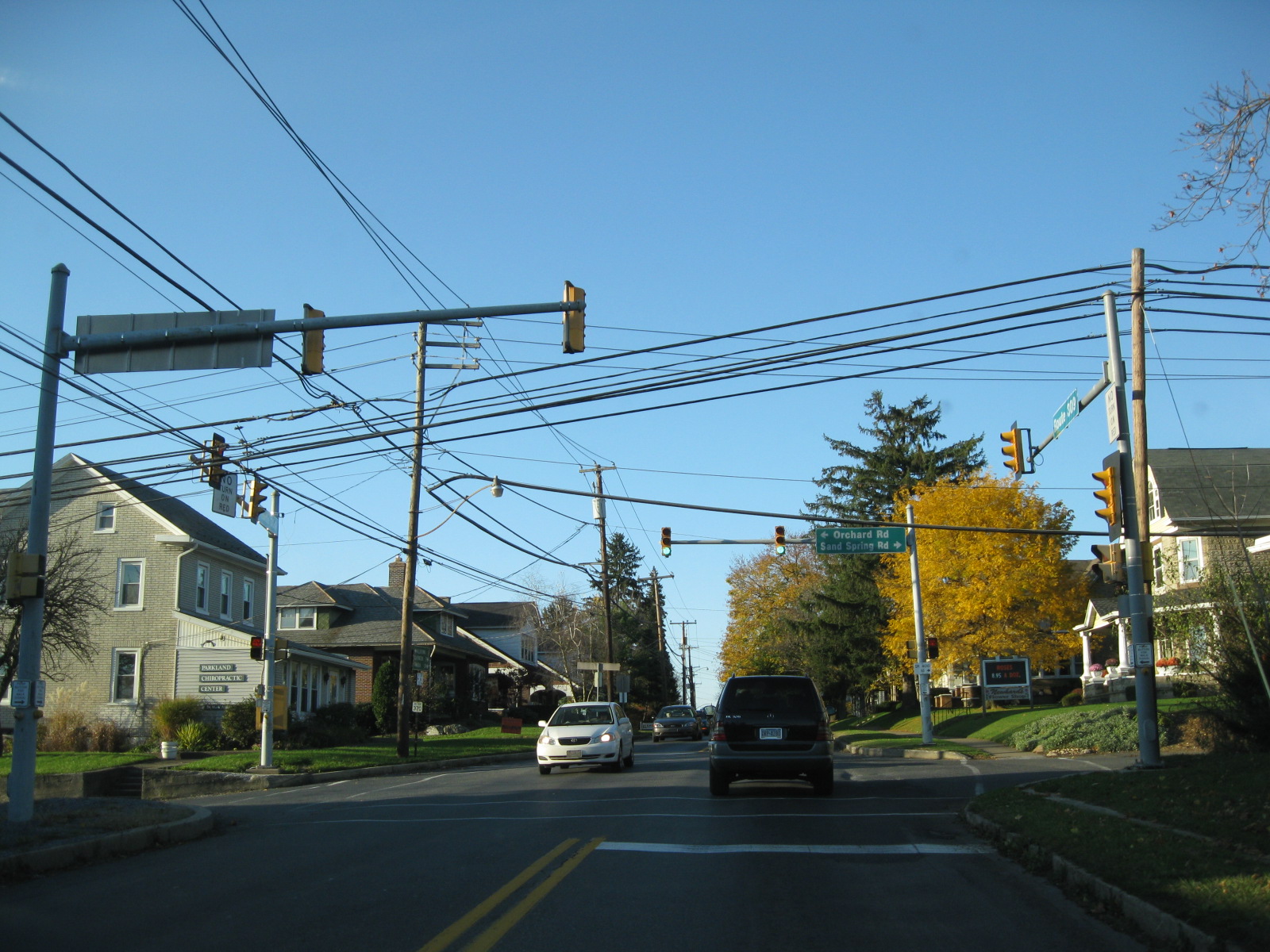A photograph captures a bustling intersection in North America, showcasing a typical suburban scene. The wide street, adorned with double yellow lines, is flanked by rows of residential houses on both sides. Several cars populate the intersection: directly ahead is an SUV, while a white car faces the opposite direction. Behind these, a compact car and a smaller green car are visible. A green road sign indicates "Orchard Road" to the left and possibly "Sandspring Road" to the right. The sky is a clear, vibrant blue, suggesting pleasant weather. Tall telephone poles with crisscrossing wires line the street. Trees, some with bright yellow leaves indicative of early fall, dot the landscape. The play of light and shadow across the scene suggests it might be morning or late afternoon, contributing to the tranquil suburban atmosphere.